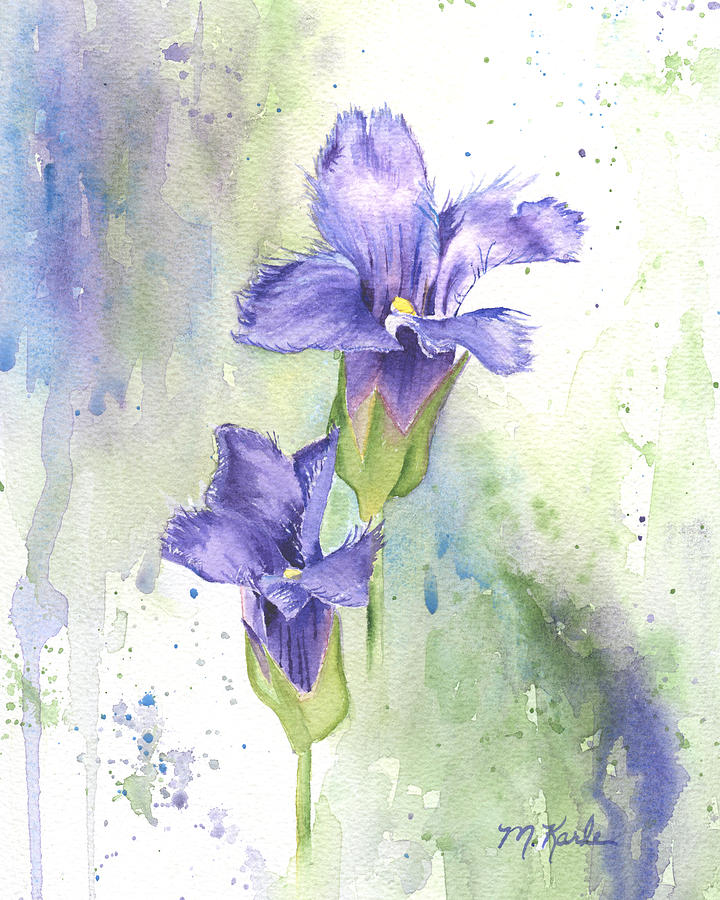The image is a detailed watercolor painting of two purple flowers in full bloom, each with four vibrant petals and a bright yellow stamen at the center. The flowers emerge from green stems and leaves, with the blooms arranged vertically—one positioned slightly higher and to the left of the other. The background is an artistic blend of shades of purple and green, featuring a mix of speckled patterns and broader paint strokes, along with some liquid-like smudges. Splashes of white dots are more prominent in the upper right corner, adding texture to the composition. The painting is signed in the bottom right corner in cursive, reading "M. CARLE" (or possibly "M.O.K.R.L.E"), anchoring the portrait-oriented artwork.